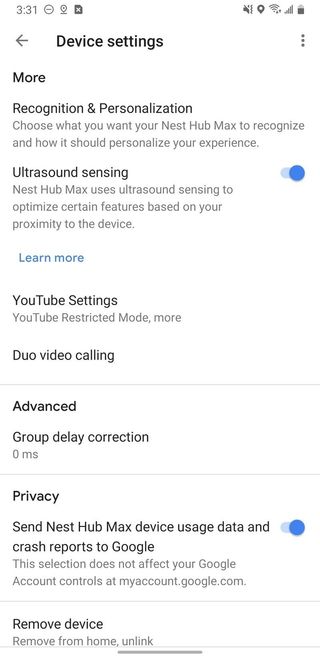The image displays the settings menu of a Nest Hub Max device, detailing various options for user customization and personalization. The menu is as follows:

- **Device Settings:**
  - **More**
  - **Recognition and Personalization:** 
    - (In smaller gray font) "Choose what you want your Nest Hub Max to recognize and how it should personalize your experience."
  - **Ultrasound Sensing:** 
    - (In smaller gray font) "Nest Hub Max uses ultrasound sensing to optimize certain features based on your proximity to the device."
    - (Indented and in blue font) "Learn more"
  - **YouTube Settings:** 
    - (In smaller gray font) "YouTube Restricted Mode, more."
  - **Duo Video Calling**
    - (Separated by a faint gray line)
  - **Advanced**
  - **Group Delay Correction:**
    - (In slightly fainter black font)

This detailed layout offers users a clear understanding of how to personalize their Nest Hub Max according to their preferences and identify the functionalities enabled by proximity detection and other advanced features.